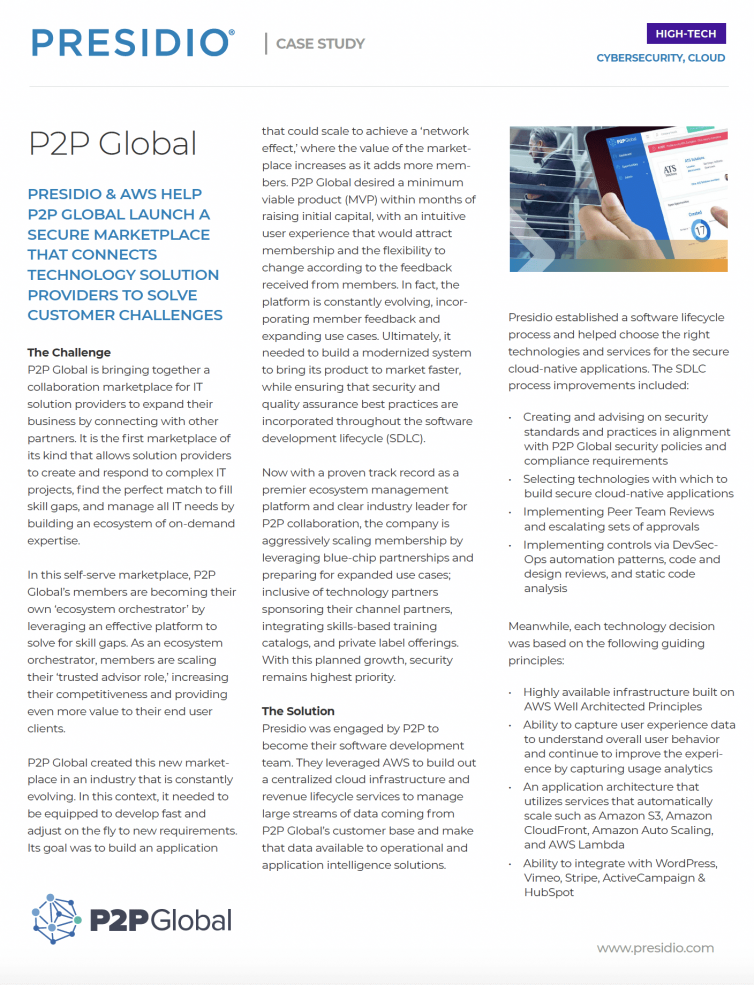**Caption:**

On this page, the top section prominently features the title "Presidio Case Study." To the right, a purple box highlights the term "Hitech," while below it, the words "cybersecurity.cloud" are displayed in striking blue font. The top left corner is marked with an informative passage: "P2P Global, Presidio, and AWS help P2P Global launch a secure marketplace that connects technology solution providers to solve customer challenges," all written in blue.

Below this passage, the text introduces "The Challenge." P2P Global aims to create a collaborative marketplace for IT solution providers, facilitating business expansion by connecting partners. This first-of-its-kind marketplace enables providers to engage in and respond to complex IT projects, find the perfect match for skill gaps, and manage all IT requirements by crafting an ecosystem of on-demand expertise. In this self-serve marketplace, members of P2P Global act as their own ecosystem orchestrators, utilizing an effective platform to address skill shortages. As orchestrators, members enhance their role as trusted advisors, boost their competitiveness, and deliver increased value to end-user clients.